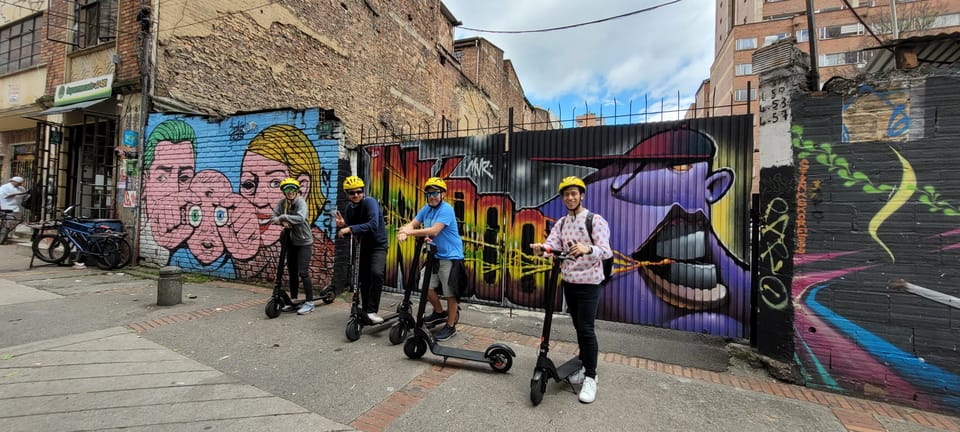This vibrant color photograph captures an urban city street, viewed in a panoramic, sideways landscape orientation. The scene is busy and detailed. The foreground features four boys standing with motorized black scooters, all sporting matching yellow bike helmets. Their attire varies, with some wearing shorts and others in black pants, some in long sleeves and some in short sleeves, adding a casual, adventurous vibe. They are positioned on a dirty cement sidewalk, suggesting they might be tourists who rented these scooters.

Behind the boys is a large wrought iron gate with corrugated tin that has been vividly painted with graffiti. This graffiti includes a purple baseball player and some words, part of the vibrant street art that characterizes the scene. To the left of the gate, a brick wall adorned with a pop-art style mural stands out. This artwork depicts a man, woman, and child with exaggerated features, including the parents holding the child's oversized blue eyeballs, creating a surreal and quirky image.

The scene is framed by old brick buildings, their facades crumbling to expose the underlying brickwork, suggesting a long history weathered by time. In the background, modern high-rise apartment buildings loom over the scene, contrasting with the old and decaying surroundings. On the left in the distance, there are bikes parked and possibly some storefronts, with graffiti and tagging extending further along the wall. A man stands on the sidewalk, adding to the bustling urban atmosphere. The photograph captures a colorful, gritty snapshot of city life, rich with artistic expression and urban decay.